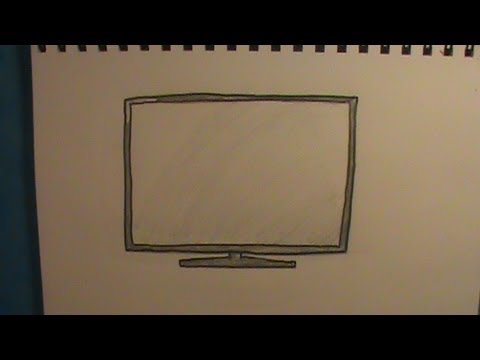The image is a detailed hand-drawn sketch of a modern flat-screen TV or computer monitor. It occupies the center of a white sketchpad, which is discernible by the spiral notebook binding visible at the top edge. The sketchpad lies flat against a predominantly black background with a slight bluish tint on the left side. The monitor is freehand drawn in pencil, with precise detailing including a thin, black border around the screen and a slender base. Noticeable shading adds dimension to the frame and base, with the upper left of the screen left white, possibly to indicate glare or shine. Some smudging within the screen area suggests an attempt to add texture, particularly towards the bottom. The clean, minimalist composition focuses entirely on the monitor, with no other elements on the page.